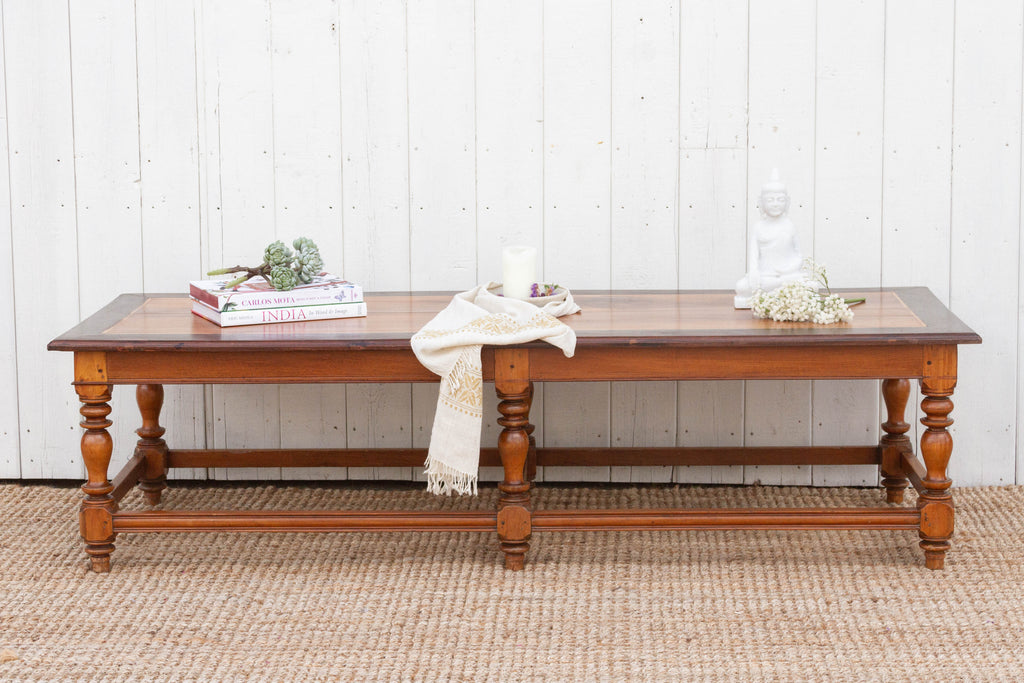This image features a medium oak-colored wooden coffee table with a darker edge stain, positioned on a light coral or pinkish throw rug. The table has a distinct structure, supported by six legs—two in the middle and two on either side to support the weight. 

In the center of the table sits a white pillar candle within a white bowl, adorned with a white scarf featuring a gold design. Surrounding the candle is what appears to be lavender. On the right side of the table is a Buddha-like statue, in front of which lies a collection of small white flowers. Additionally, the table holds two books: one titled "India" and another by Carlos Mota, though the title is not clearly visible. Atop these books are decorative elements resembling hens and chick plants.

The table is set against a background of a white-painted wooden panel wall, adding a rustic charm to the scene.